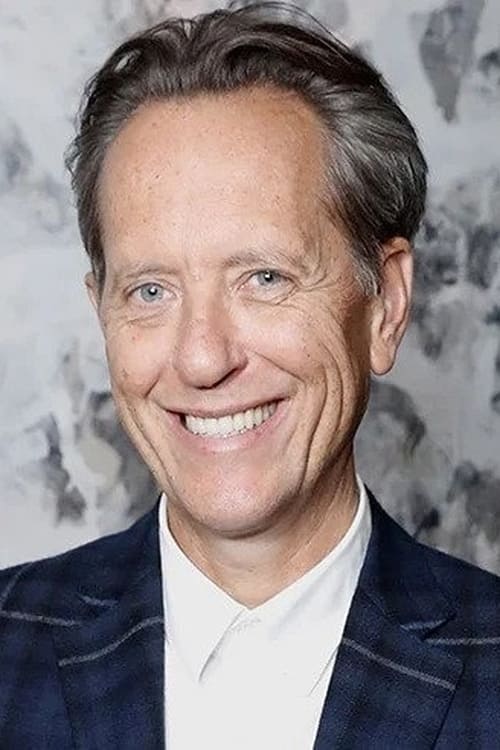This color photograph is a close-up headshot of Richard Grant, a distinguished older gentleman who appears to be around 60 to 65 years old. Richard, a Caucasian male, is smiling broadly at the camera, showcasing the lines and wrinkles around his mouth and crow's feet near his eyes. His hair, predominantly gray but with hints of brown, is neatly combed back, highlighting his large forehead and striking icy blue eyes.

He is dressed in a stylish blue suit jacket adorned with thin white stripes, giving it a plaid appearance. Beneath the jacket, he wears a plain white button-down shirt with the collar open, adding to his relaxed yet sophisticated look. The backdrop of the photograph features a gray marble texture with a mix of white and dark gray hues, lending an elegant atmosphere to the image.

However, the photo quality is somewhat compromised; it is low-resolution and suffers from JPEG artifacting, indicating it has been heavily compressed over time. Despite this, Richard's warm, happy demeanor remains the focal point of the image.